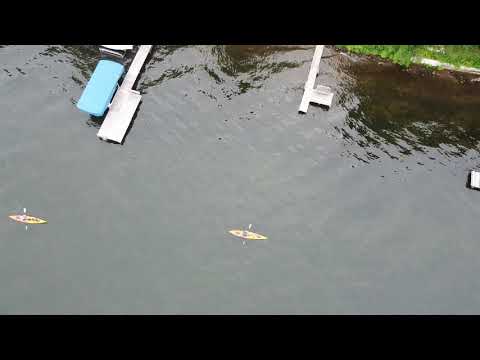This digital aerial photograph, framed with black headers and footers, captures a daytime scene looking straight down onto a calm, dark brown river. The river is largely still, devoid of white-capped ripples, and is navigated by two yellow kayaks equipped with white oars. The kayaks are spaced in a single file line, with the left kayak closer to the image's edge and the right one near the center. The kayakers themselves are difficult to distinguish due to the high vantage point. In the top right corner, patches of green shrubbery are visible, along with two white piers extending from the shore. The left pier is longer and features a blue-roofed section with a boat moored beside it. Overall, the photograph beautifully captures the serene river setting, dotted with kayaks and bordered by lush greenery and piers.